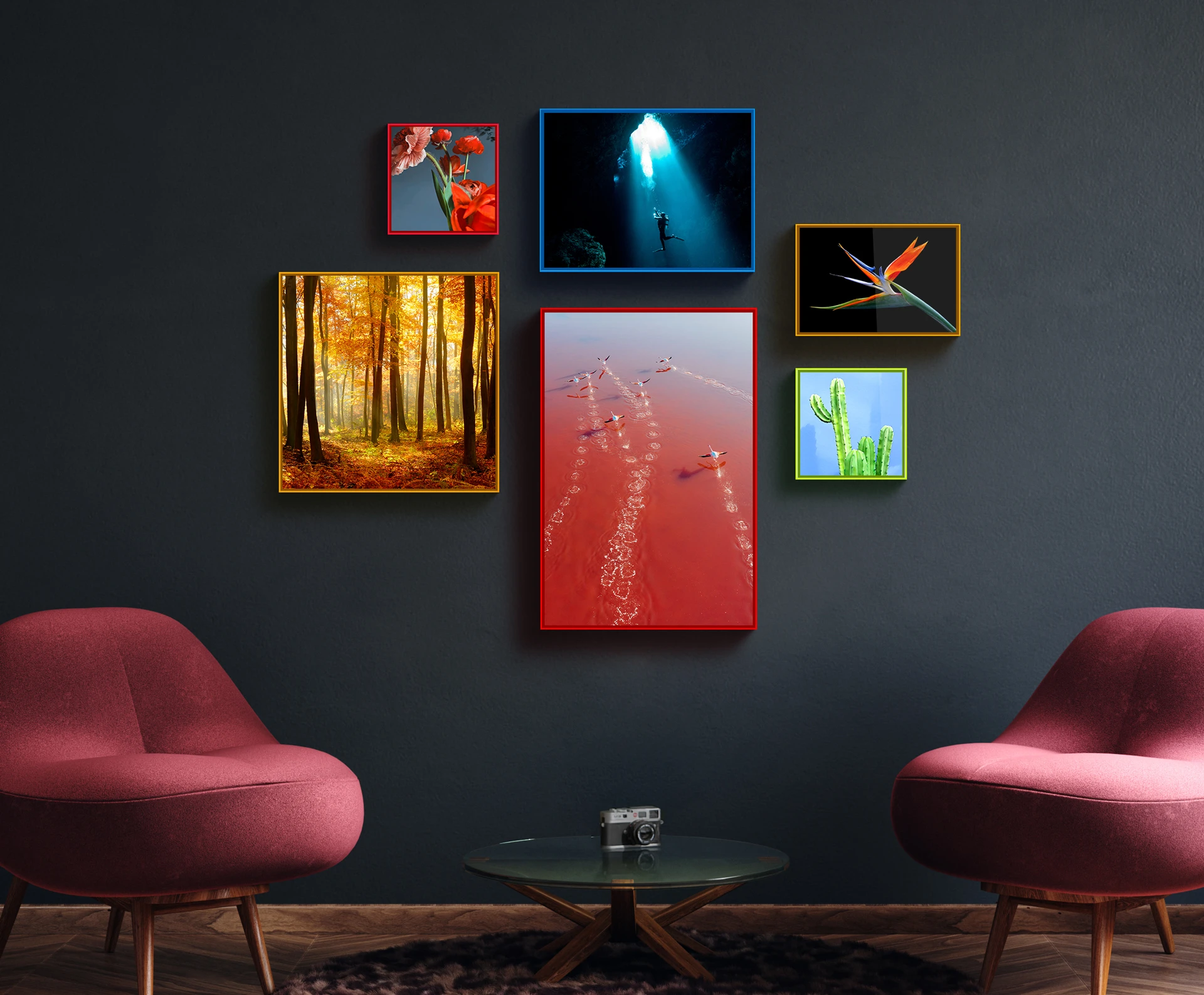The room features a slate matte-textured wall, giving it a dark grayish-blue appearance, which serves as the backdrop for a collection of six photographs in various colorful frames. The photographs include a red-framed image of red cranes, a gold-framed woodland scene with yellow leaves on the far left, a blue-framed picture of a diver swimming toward the surface, a yellow-framed portrait of a bird of paradise flower, a green-framed shot of a cactus against a blue sky, and a large square red-framed photo of red sand.

Beneath these vivid images, the floor is made of hardwood, lending a warm contrast to the dark wall. At the center of the room is a round leopard-skin patterned rug, perfectly anchoring a coffee table with light wooden legs and a round glass top. A camera rests atop this table, adding a touch of personal or artistic character.

Flanking the table are two plush chairs, designed without armrests and featuring minimal backrests. These chairs are primarily wooden with light wood seats and legs, but they boast thick, upholstered cushions in a striking reddish color, providing both style and comfort to the room. The overall setting is completed by the careful placement of these elements, creating a balanced and inviting atmosphere that could be part of an apartment or a sophisticated waiting room.